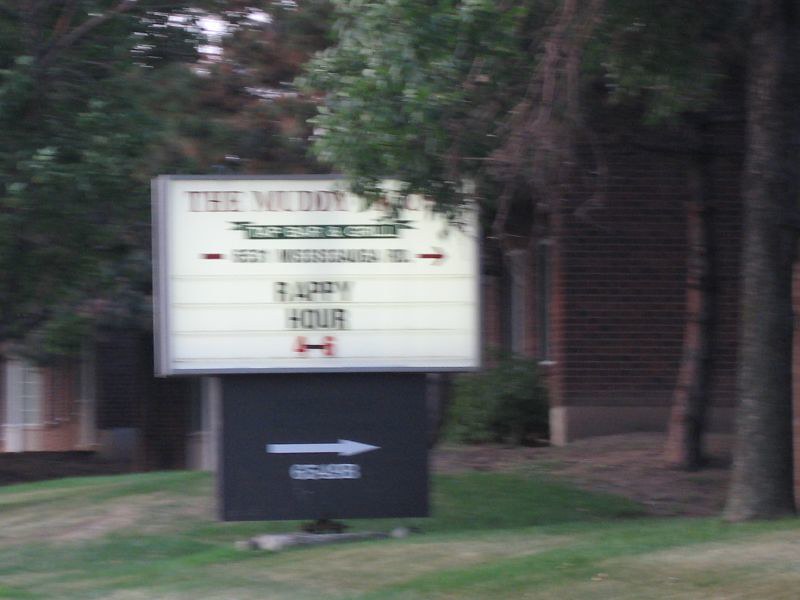The photograph captures an outdoor setting featuring a grassy area with scattered patches of dirt. In the background, a mix of thick and thin tree trunks with varying shades of brown can be seen, along with dense, dark green foliage. Central to the image is a somewhat blurred sign with a white and silver frame, partially obscured by a leafy branch. The sign prominently displays "The Muddy," followed by partially covered text that reads “tap bar and grill.” Below, it announces "happy hour 4 to 6" with a directional white arrow pointing to the right, above a black panel listing some numbers. Surrounding the sign is a yard-like area with grass that is greener in some patches and brown in others. At the base of the trees, patches of dirt are visible, and in the backdrop, the brick walls of a building peek through the foliage, adding a rustic touch to the scene.